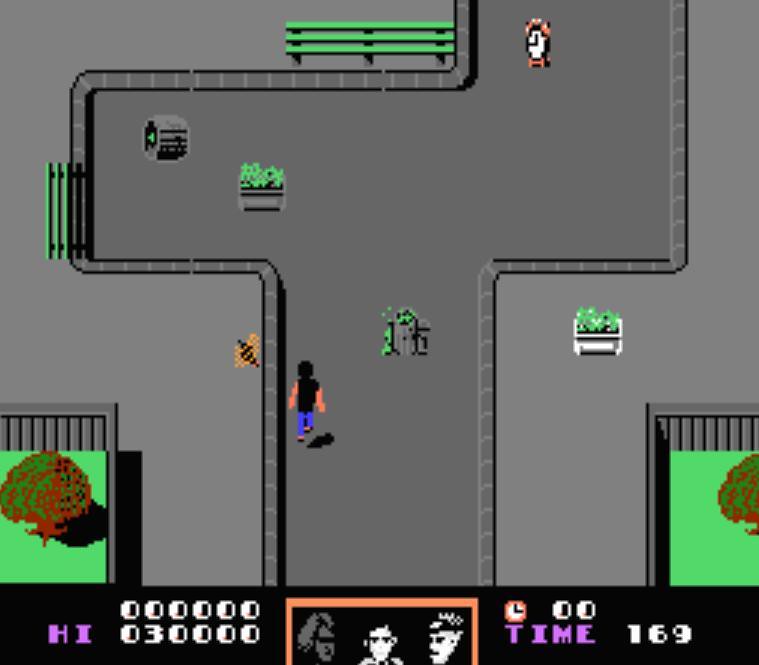The image appears to be from a video game and depicts a scene featuring a variety of elements within a predominantly grey landscape. Central to the composition is a green bench situated at the top center. To its immediate right is a clock icon, characterized by an orange top and bottom, a white clock face, and small black hands.

Below the clock, there is an image of a potted plant with a white pot and green leaves, indicating its foliage. Moving towards the bottom right from the plant, a small grassy area is enclosed by a grey fence. In this area, an obscured tree image, rendered in shades of brown and orange, is visible.

Close to the center, another icon displays a grey and green color scheme. Below this, to the left, is an image of a person. The figure has a black body, tan arms, blue jeans, tan shoes, and casts a small black shadow.

In the upper left, there is an image resembling a bee with characteristic orange and black stripes. Directly below this bee, there is another grassy area and a tree icon, also situated behind a grey fence. Numerous green benches are scattered throughout the scene, adding to the overall green motifs against the grey landscape.